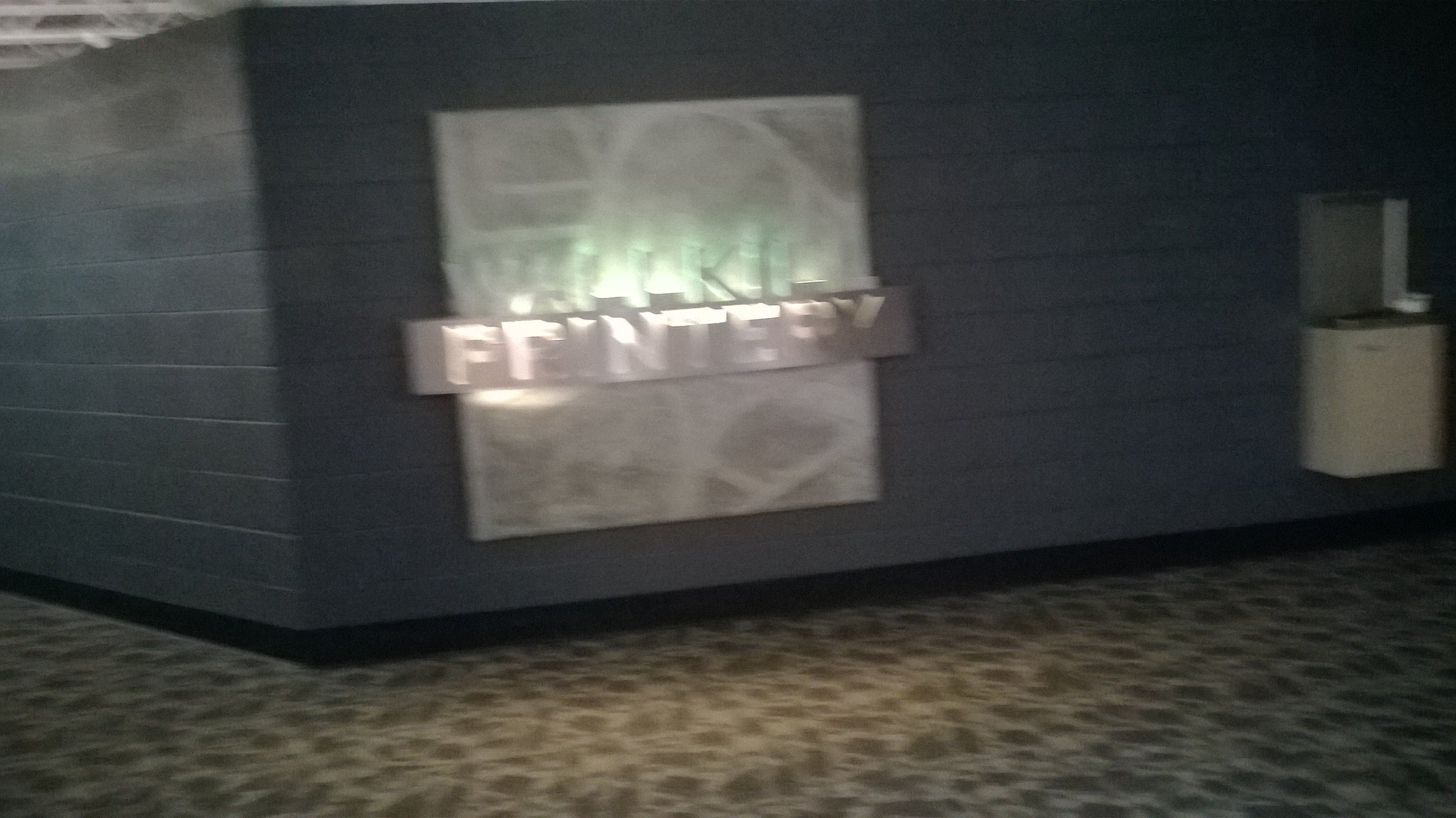The image showcases a video game snapshot of the interior corner of a building, possibly mimicking a nightclub entrance or a trendy modern setting. The composition is roughly one and a half to two times wider than it is tall, with a walkway slanting diagonally to the left and another extending horizontally. Dominating the scene is a dark brown cinder block wall adorned with a large decorative silver square plaque resembling a window. This plaque features a semi-reflective, milky white swirl design and a centrally placed rectangular banner illuminated with the word "Printery," though some letters are partially cut off. Above this banner, faded text is barely discernible. The baseboard along the bottom of the wall is black. To the far right, a beige drinking fountain nestles against the wall. The floor is covered in a leopard print carpet in shades of brown and beige, adding a touch of wild texture to the scene. A small patch of ceiling is visible, hinting that the room might be in a basement, further contributing to its mysterious, nightclub-like ambiance.